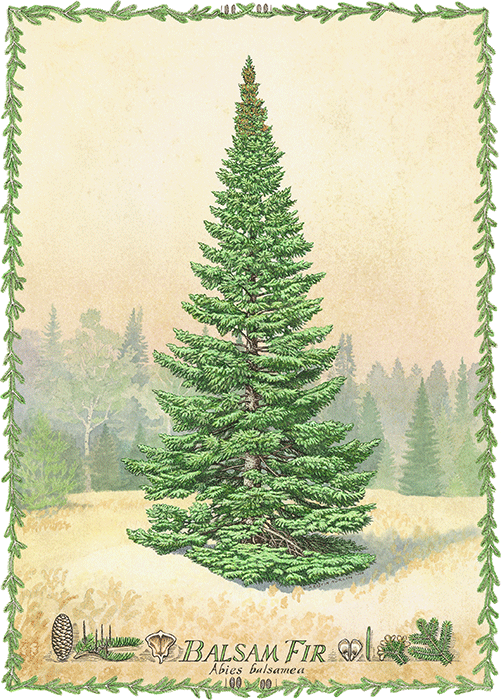This detailed illustration presents a beautifully shaped balsam fir tree, characterized by its wide base narrowing gracefully towards the top. The tip of the tree shows a hint of brown, possibly indicating pine cones. The tree stands prominently in the center, with its trunk slightly visible through the lush branches, reminiscent of a classic Christmas tree. The image is artistically framed with a delicate border of balsam fir branches and needles, enhancing its vintage and festive appeal, suitable for a Christmas card.

The background features a variety of trees in lighter, blurred shades of green, creating a subtle contrast that emphasizes the central fir tree without detracting from it. The ground appears tan and dried, suggesting a winter setting. The lower part of the image includes detailed illustrations of balsam fir needles and a pine cone, along with the text "Balsam Fir, Abies balsamea." The text adds a scientific touch to the artwork, pairing beautifully with the realistic and intricate depiction of the foliage.